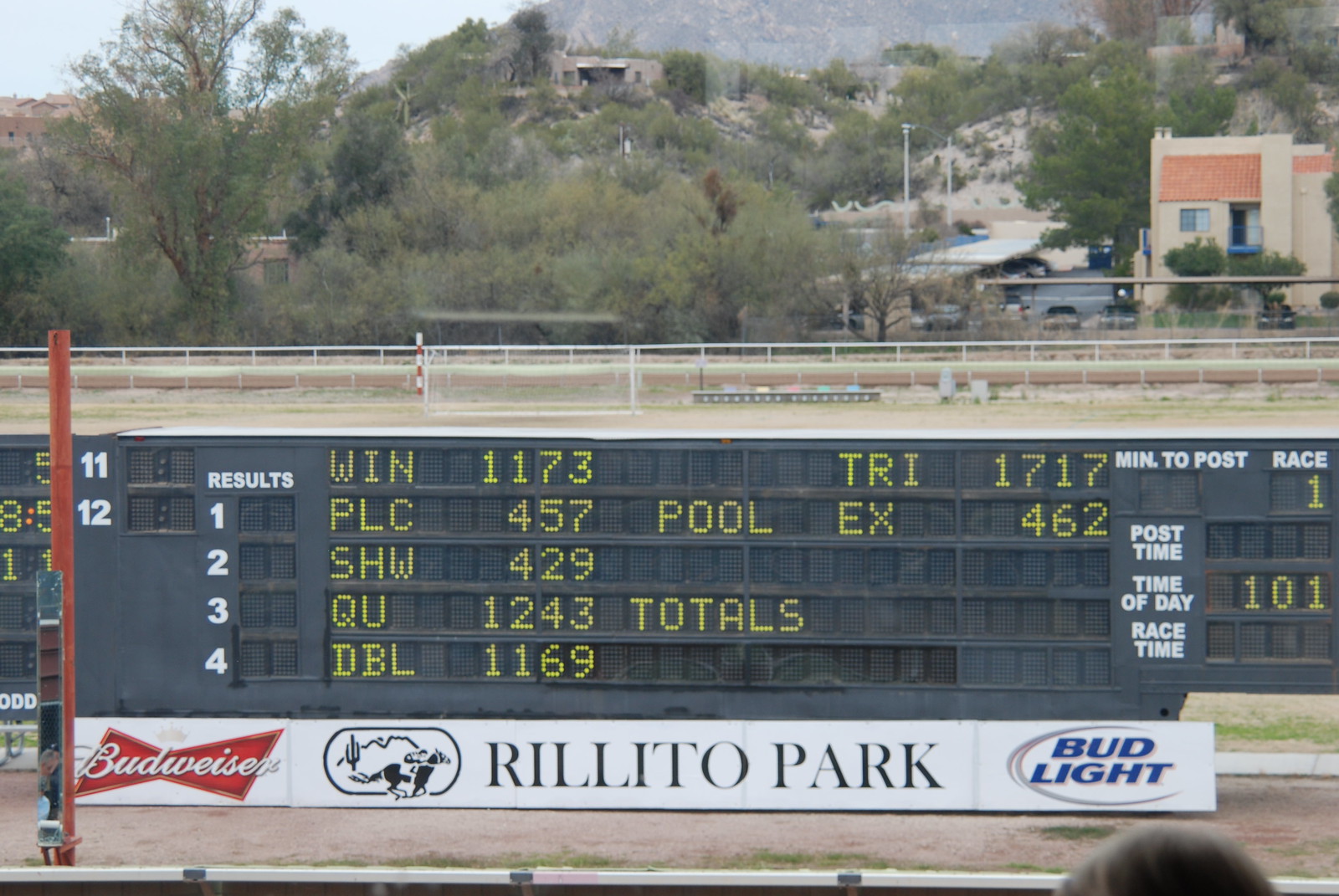This color photograph, taken outdoors, prominently features a very large digital scoreboard, likely at a racetrack, possibly for horse racing. The scoreboard displays race results in large, clear text: at the top, it reads "WIN-1173," "PLC-457," "SHW-429," "QU-1243," "DBL-1169," "TRI-1717," and "EX-462." Near the bottom, there are advertisements with the Budweiser and Bud Light logos, along with "Rillito Park" clearly spelled out. The background reveals a picturesque setting with a mountain, trees, and a building behind a cyclone fence and possibly a barrier for the track.